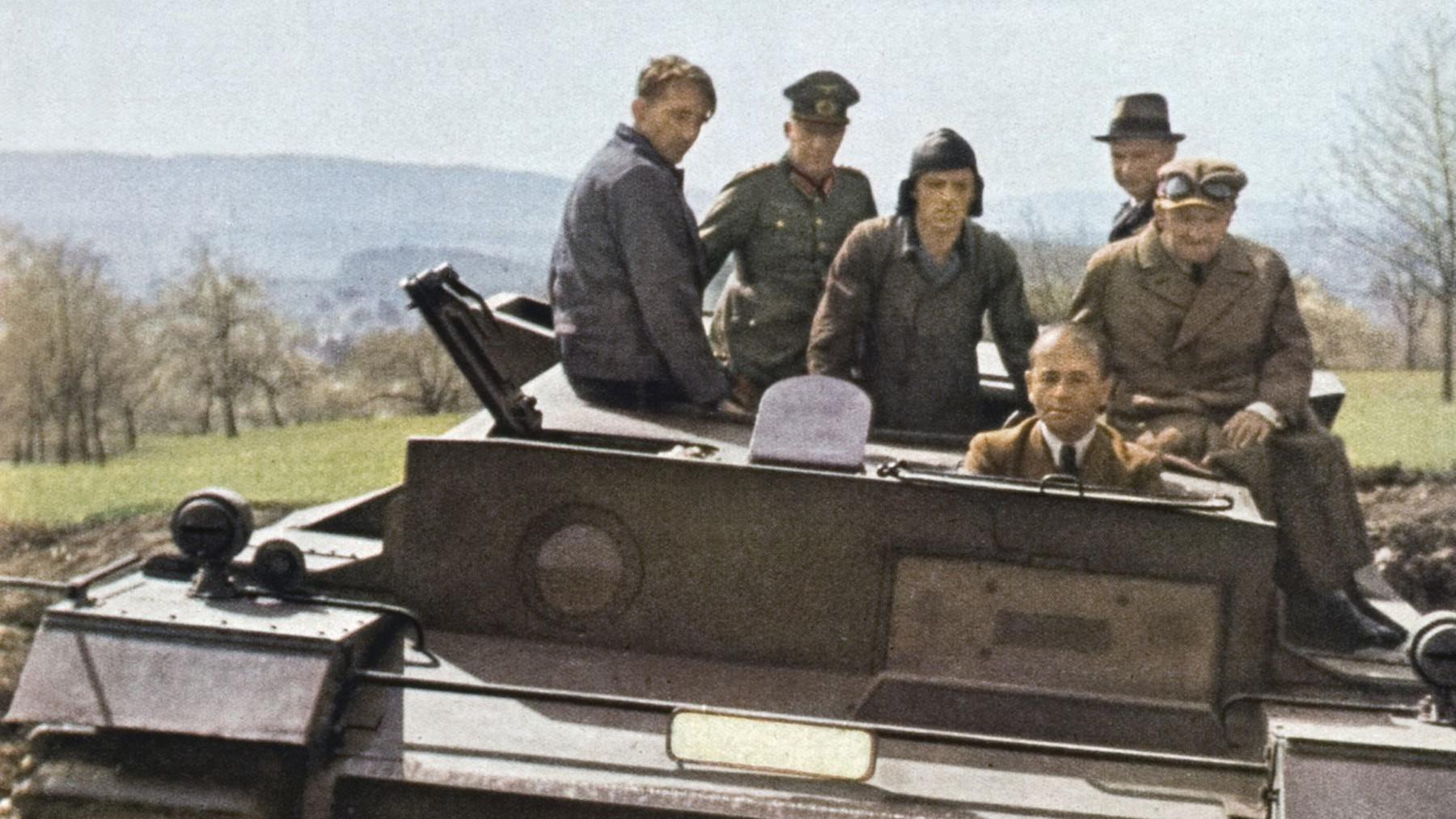The image depicts a group of six men, seemingly captured in a photograph from the first half of the 20th century. They are positioned on top of what appears to be a war tank. The photograph is grainy, reflecting its age, yet the men and the background are discernible. Four or five of these men are dressed in military uniforms, indicative of soldiers, while one man, centrally located, is distinguished by his brown suit and black tie, standing out without any military attire. 

The men vary in age, with some appearing to be in their 20s or 30s, while others look to be in their 50s or 60s. Among them, an older gentleman is notable; he wears a golf cap, sunglasses, and a raincoat, sitting on the tank with his arms resting on its edge. Another man dons a gray derby and a fedora, paired with a dark suit.

The backdrop features elements of nature: green grass, trees, distant mountains, and a clear blue sky. The photograph is dominated by neutral colors like black, white, gray, tan, and brown, but also includes other hues such as blue, yellow, and green, enhancing its overall composition. All six men gaze directly into the camera, reinforcing the photo's engaging and direct nature.